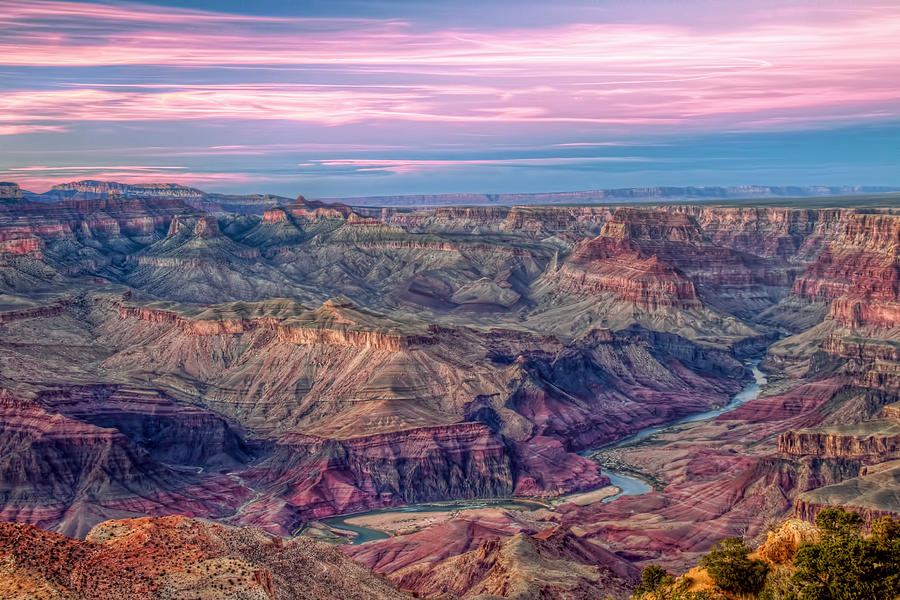This is an aerial photograph of a colorful, mountainous valley likely part of the Grand Canyon, captured around sunset or early morning. The photograph is highly detailed, showcasing tall and deep canyons with very distinct geological layers that have been carved out by a small, winding river at the bottom. The canyon walls display a vivid palette of red, purple, brown, pink, and black sediments, highlighting thousands of years of natural history. Large plateaus perched atop the canyon contribute to the dramatic landscape, emphasizing the high altitude from which they were cut. The sky, occupying the upper third of the photograph, is a stunning array of pale grey-blue, light pink, dark pink, mauve, electric pink, and white, reflecting down and casting an ethereal glow on the rock formations.

In the foreground, the details become even more vivid, with dark, shady sand, orange hues, and what appears to be a shrub in the bottom right corner. The river meanders gracefully from the right-hand side, flowing towards the left, bending and reflecting the sky's colors. The interplay between the sky and the canyon creates a surreal, almost painting-like quality, making the image extraordinarily vibrant and captivating.